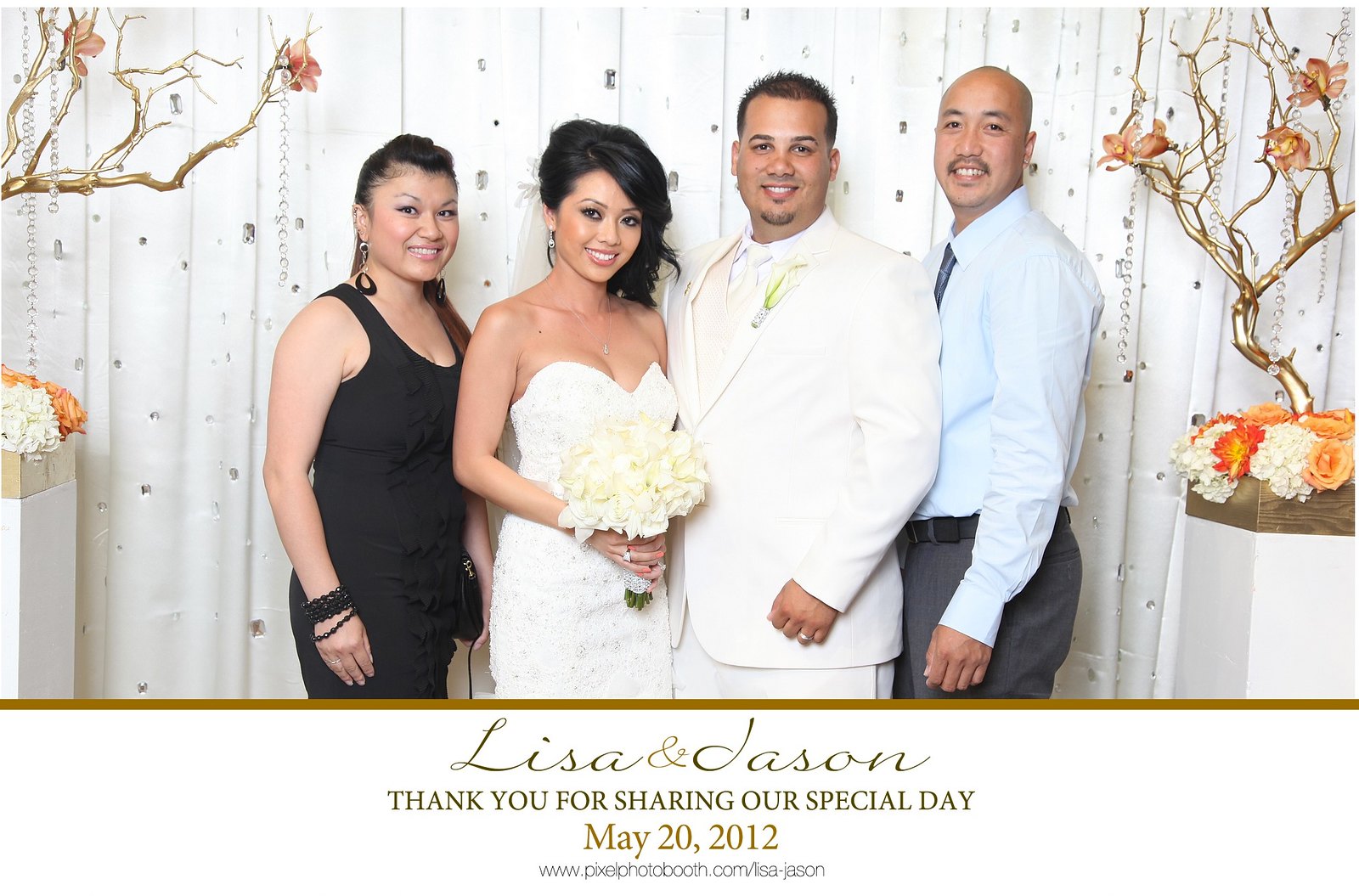This detailed wedding photo features the bride and groom at the center, flanked by two attendants. The background showcases an elegant off-white curtain adorned with stylized golden tree branches and lightly colored flowers in shades of white, pink, and light orange. Dangling chains or ornaments are visible, adding a touch of sophistication. At the bottom of the photograph, a gold line with cursive text reads, "Lisa and Jason," followed by the message, "Thank you for sharing our special day, May 20th, 2012," and the small print of "pixelphotobooth.com."

The bride, an Asian woman with long, flowing black hair, wears a strapless white dress and holds a bouquet of white flowers. The groom stands beside her in an all-white suit, white pants, and a white tie, his light tan complexion complemented by short, spiky brown hair and a thin goatee. To their left is a bridesmaid in a black dress, adorned with black jewelry and looped earrings, with long brown hair. To their right is the best man, wearing dark gray slacks and a light blue buttoned-up shirt. He is bald with a mustache. This beautifully staged photo captures the essence of Lisa and Jason's wedding celebration.